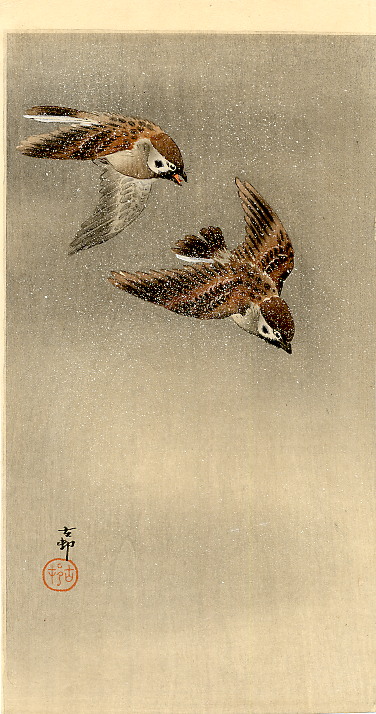This painting, which is taller than it is wide, features two variegated brown birds flying against a mostly grayish, cloudy sky that fades to lighter shades with waves of white. Both birds, resembling sparrows, are primarily variegated brown with patches of black on their upper wings, and their underbellies and the undersides of their wings are whitish gray and light brown. Their heads are deep brown with a white facial mask and black markings beneath. The bird on the right is diving downward with fully extended wings, showing brown with black spots on the upper side and darker gray on the underside. Its tail is fanned out, and it has a short, pointed yellow beak with white around its black eyes. The bird on the left also seems to be descending, with its wings in a downward position, showing the brown upper side and the white underbelly. Its tail is more closed, and its beak is open, revealing a hint of red inside. The background is an abstract composition featuring pale yellowish, tan, and grayer hues. In the lower left-hand corner, a red circle contains red Japanese characters, with black characters above it.